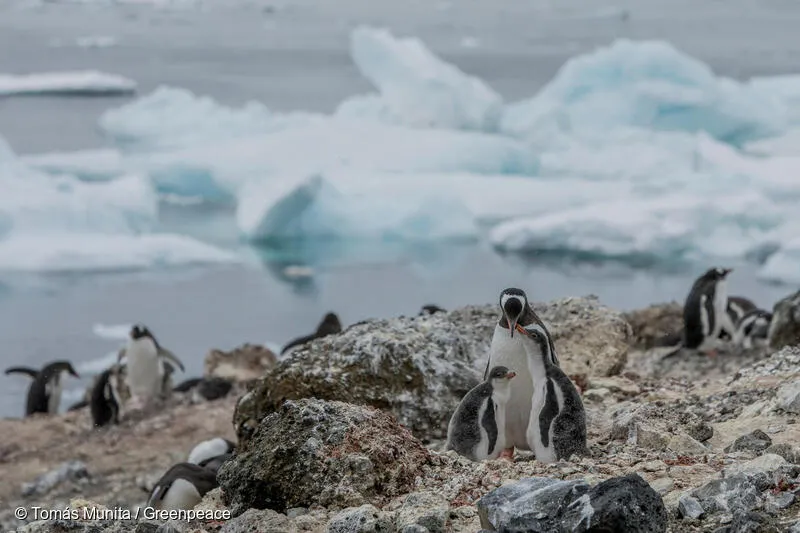In a breathtaking photograph by Tomas Munita for Greenpeace, a group of penguins of various shapes and sizes, yet all of the same species, are scattered across rugged, grayish-brown rocks in the foreground. The focal point is a mother penguin standing prominently towards the camera with her head tilted down, flanked by two young penguins. The one on her right, slightly shorter, has its beak reaching up towards her, while the smaller penguin on her left faces sideways. In the background, additional penguins are visible—some walking with their wings outstretched, others facing different directions. The distant scenery reveals a dramatic Antarctic landscape, featuring blurred, floating blocks of ice and glaciers atop the water, extending to a desolate sea. This striking image captures the unique environment of Antarctica, with the stark blacks, whites, and grays of the penguins and their rocky habitat contrasting sharply against the icy blue waters and white glaciers beyond. The bottom left corner of the image carries the photographer’s credit, "Tomas Munita / Greenpeace."